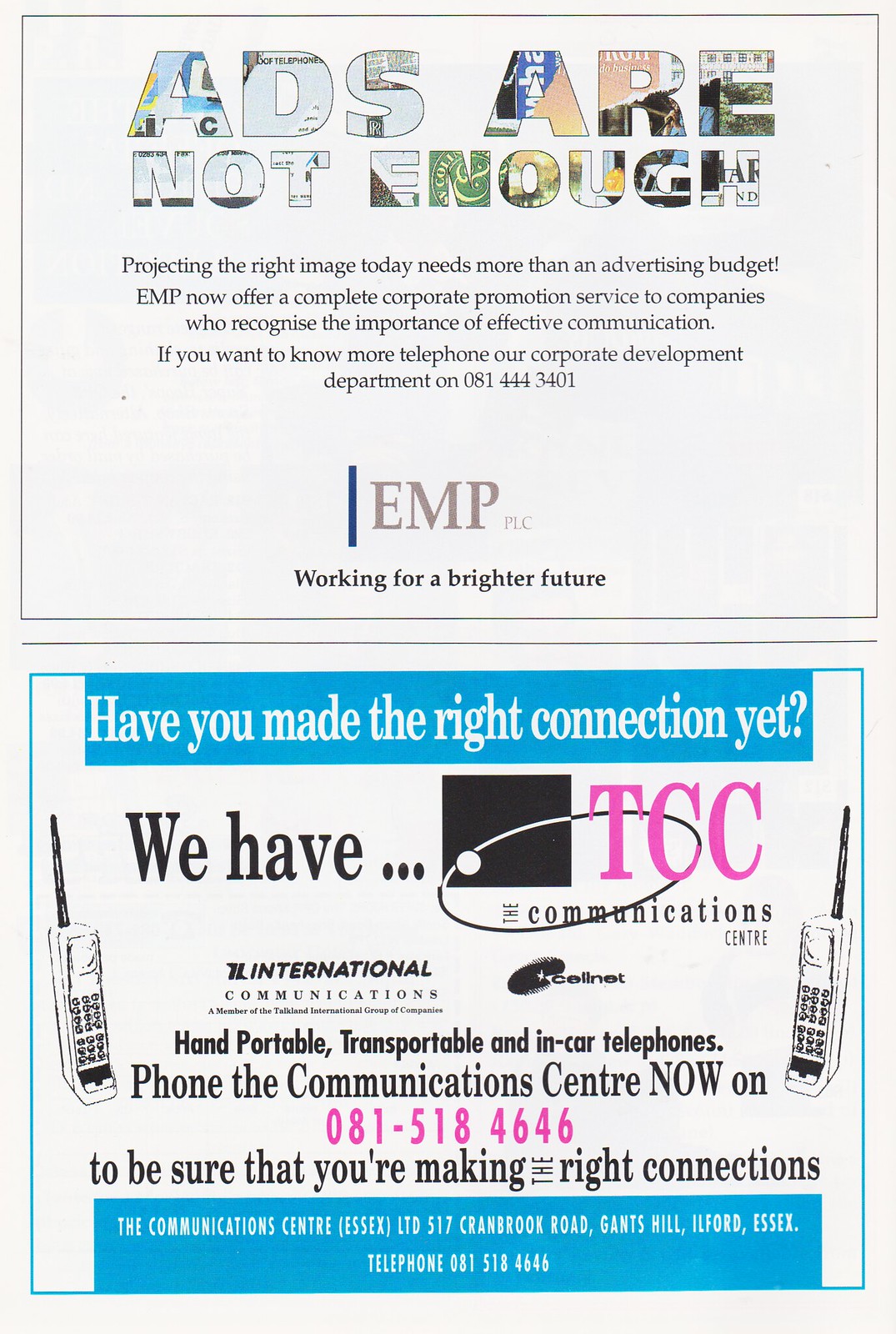This magazine page features two stacked advertisements. The top ad is set against a white background with a black outline. At the top, in colorful print, it declares, "Ads are not enough." This is followed by a paragraph explaining that effective communication today requires more than just an advertising budget. The ad promotes EMP PLC's comprehensive corporate promotion services for companies that value effective communication. The text includes a call to action with the phone number 081-444-3401. At the bottom of this section, it says, "EMP PLC, working for a brighter future."

Below this, a second advertisement is outlined in blue. The top part of this ad features a bold blue banner stating, "Have you made the right connection yet?" It introduces TCC Communications, advertising their range of old-school cellular phones, including hand portable, transportable, and in-car phones. Adjacent to images of 1980s blocky cell phones, it urges readers to contact the Communications Center at 081-518-4646. The ad concludes with another blue banner at the bottom, detailing the company's contact information: The Communications Center, Essex Limited, 517 Cranbrook Road, Giants Hill, Hillsford, Essex, and the same phone number, 081-518-4646.

Together, these ads emphasize the theme of modern connectivity and corporate communication, blending colorful and detailed text with visual elements to engage the reader.